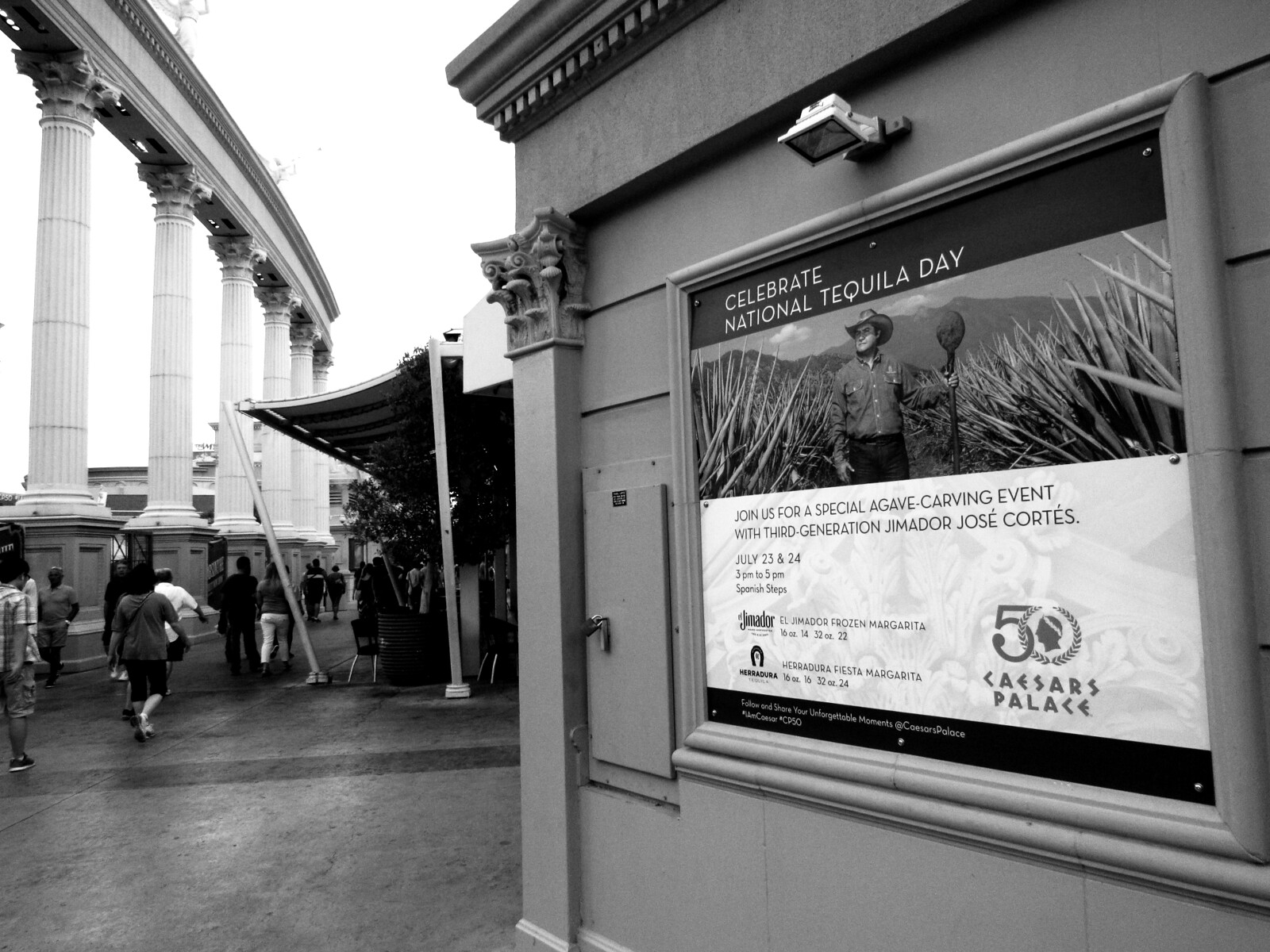This detailed black and white photograph captures an external view of a building with classical architectural elements. The building, reminiscent of structures seen in Rome or Greece, features meticulously designed columns on its left, supporting a line without a roof, creating a resemblance to the Colosseum. In the forefront, people are casually walking back and forth along the street.

Central to the image is a prominently displayed framed poster on the side of the building, celebrating National Tequila Day. The poster is headlined with "Celebrate National Tequila Day" and includes a photograph of a cowboy or farmer, donning a hat and a button-down shirt with black jeans, standing amid agave plants. He holds an iron rod, possibly a staff, surrounded by agave spikes.

Below the image, the poster invites viewers to "Join us for a special agave carving event with third generation Hemador Jose Cortez" at Caesars Palace. Additional details, such as the date and time of the event, are printed in smaller text. In the lower right corner of the poster, the logo commemorating the 50th anniversary of Caesars Palace is visible. Above the poster, a security camera or light fixture leans downwards, enhancing the visual credibility of this notable location in Las Vegas.